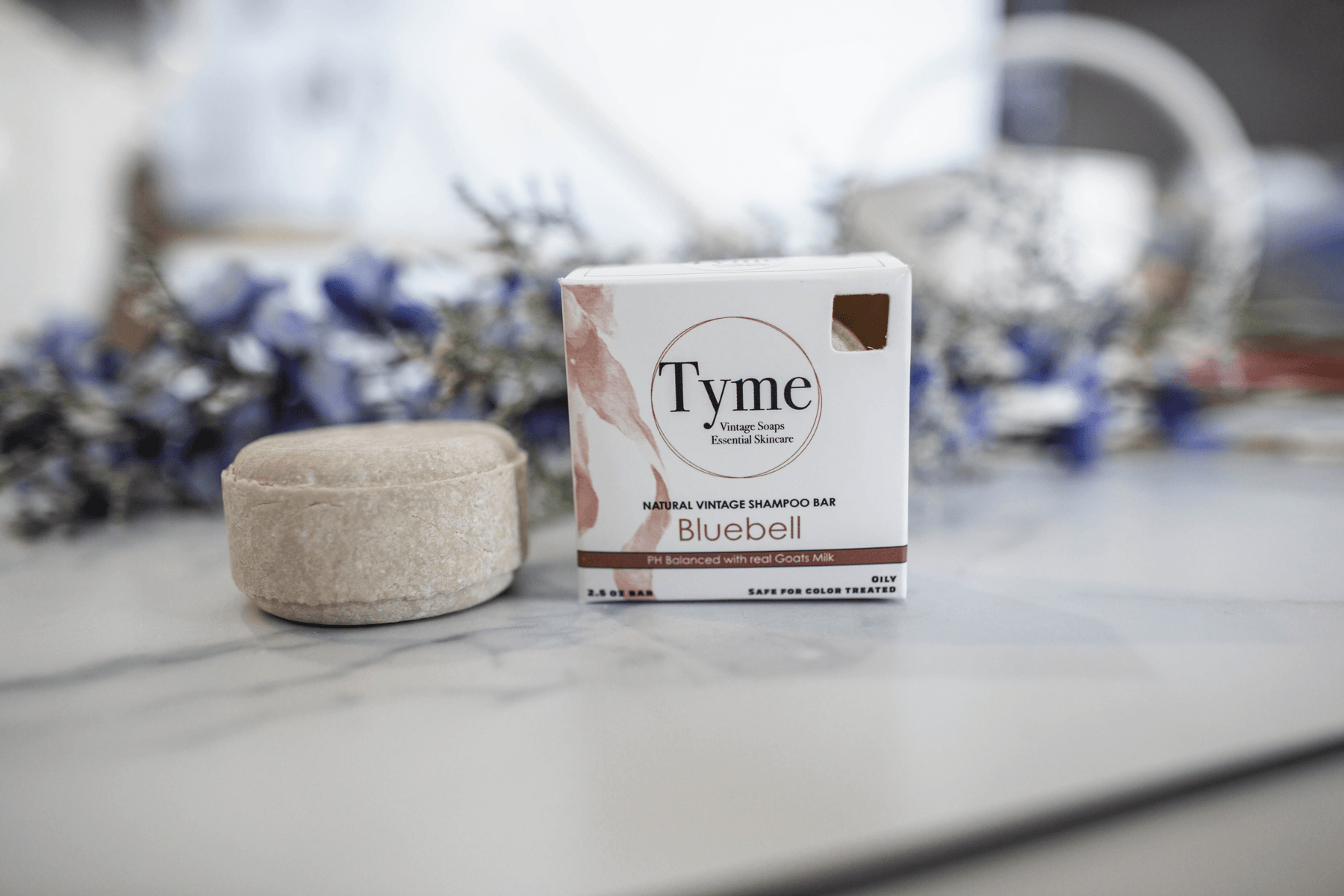This is a detailed photograph featuring a beige, round shampoo bar on the left and its packaging on the right. The packaging is a box predominantly white with brown accents and black lettering. The brand name "TYME" (T-Y-M-E) is prominently displayed at the top, followed by "Vintage Soaps Essential Skin Care" in a circular design. Below this, it reads "Natural Vintage Shampoo Bar" and "Blue Bell" in black and brown lettering, respectively. Further down, a brown banner features "pH Balanced with Real Goat Milk," and the box specifies "2.5 ounce bar" on the lower left and "Oily Safe for Color Treated" on the lower right. The items are placed on a gray to white marble countertop, which adds a subtle elegance to the setting. The background is out of focus but reveals a hint of lavender-like purple flowers and possibly a light source, indicating a window. The overall composition is slightly crooked, adding an organic, candid feel to the image.